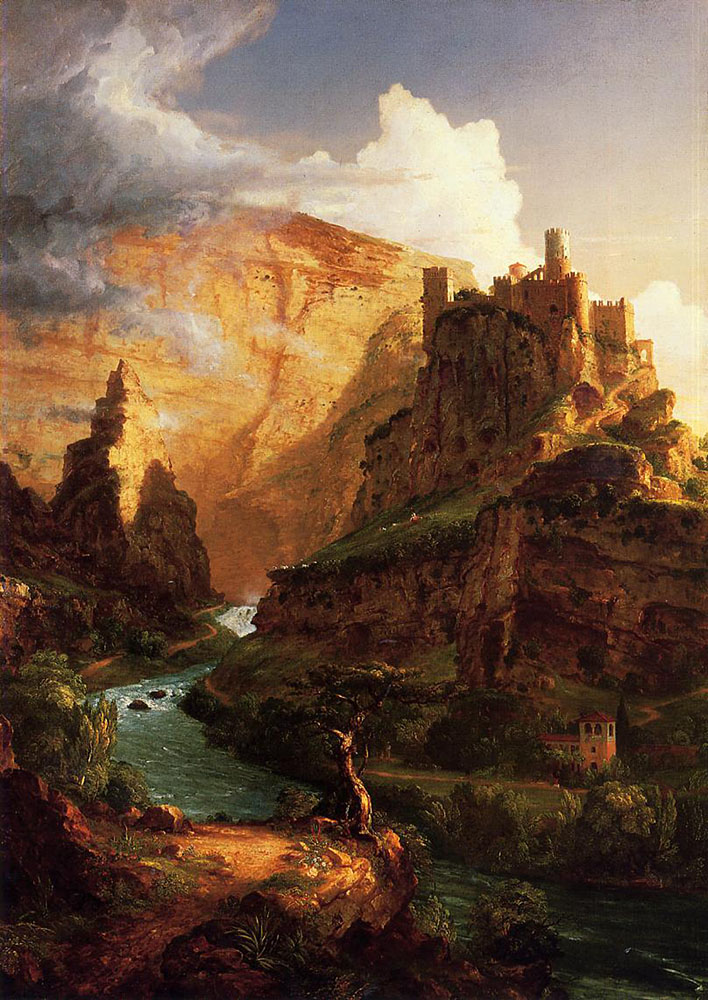This painting depicts a dramatic canyon scene, likely inspired by an Italian landscape, where a river or stream meanders through towering, rocky cliffs. The mountains are a striking reddish-orange, with hints of green vegetation clinging to the edges. The sunlight, piercing through a hazy sky filled with white fluffy and grey storm clouds, bathes the rocky terrain in a warm yellowish-orange glow, indicating a sunrise or sunset setting.

In the lower right corner, a small, two-story building with a red tiled roof and white walls stands out. The building features archway windows and is set against the backdrop of a large hill, which hosts a castle built directly into the hillside, emphasizing the historical Italian influence. Trees sprout along the riverbanks, adding a touch of green to the otherwise arid landscape.

Whitecaps dot the surface of the river, a bluish-green ribbon winding through the scene, bordered by large boulders and stones. In the lower-left foreground, a solitary tree on a landing provides balance to the composition. The sky's blend of bluish and pink hues adds to the painting's serene and atmospheric quality, capturing the tranquil yet majestic essence of the canyon.